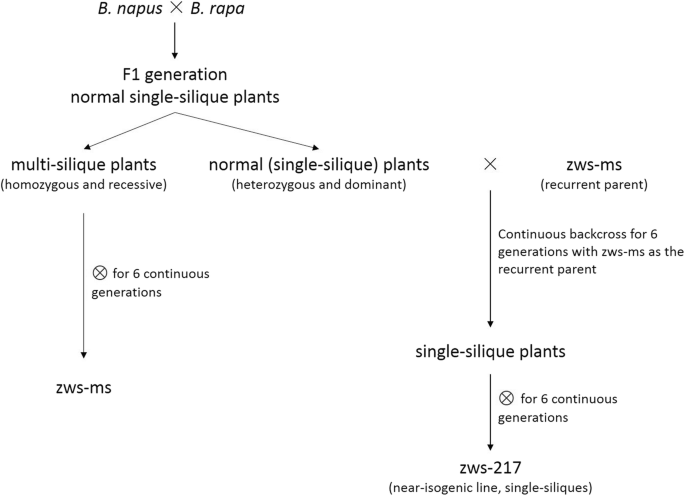The image depicts a detailed scientific chart, likely extracted from a science book or journal. It features a white background with black text and arrows, primarily focusing on plant genetics. At the top, the chart initiates with "B. napus × B. rapa," signifying a cross between two plant species. This leads to a section labeled "F1 generation normal single silique plants." From here, two arrows branch out: one pointing to "multi-silique plants" annotated as "homozygous and recessive," and another to "normal single silique plants" denoted as "heterozygous and dominant." A subsequent arrow directs to "ZWS-MS." On the right side, "ZWS-MS" recurs, with an arrow indicating a continuous backcross process for six generations, using ZWS-MS as the recurrent parent, leading to "single silique plants." The chart includes further details and numerical markers, such as "ZWS-217," indicating a near isogenic line of single silique plants. This chart serves as a genetic flowchart for classifying and understanding the hereditary patterns in specific plant species, particularly for scientific or educational purposes.